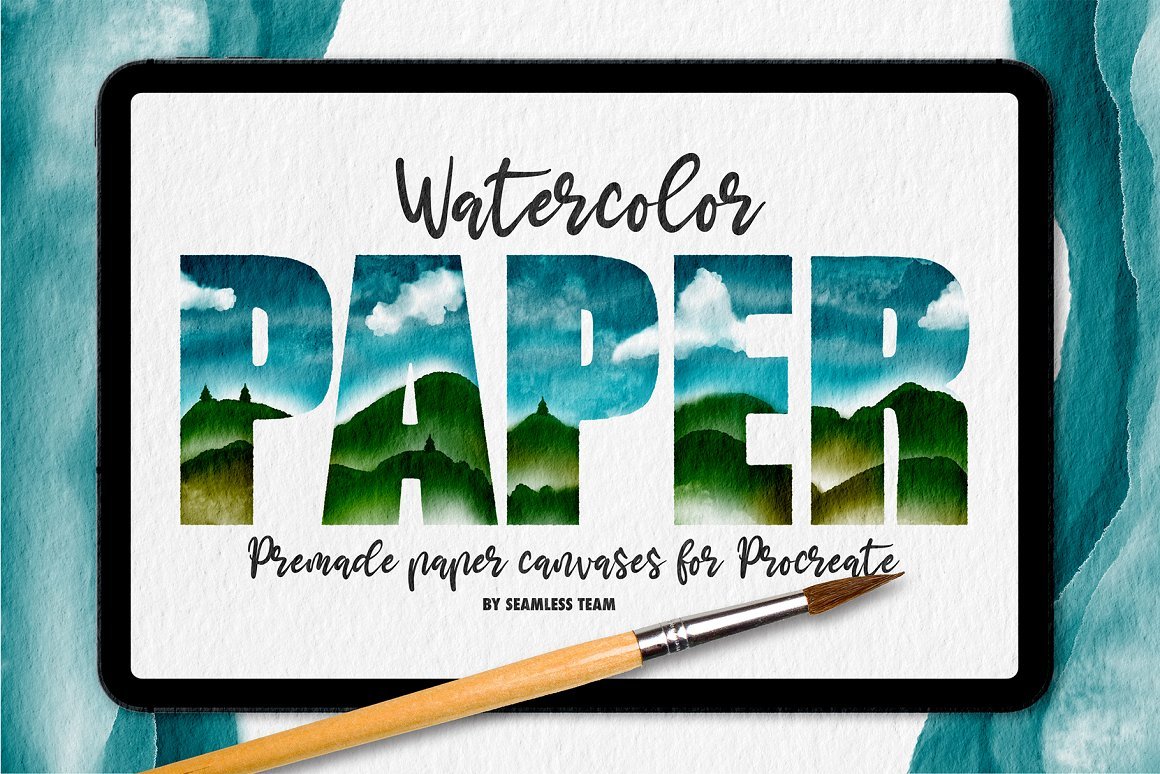The image is an artistic advertisement designed to resemble a digital drawing. It features a black rectangular frame resembling an iPad or tablet, inside of which is a sheet that displays the phrase "watercolor paper" in an artistic, handwritten style. The word "watercolor" is written in black cursive at the top, while "paper" is prominently featured below in larger, colorful letters. Each letter in "paper" is painted to depict a vibrant landscape scene: the tops of the letters showcase blue skies with clouds, transitioning to green hills at the bottom, some of which include tan-colored slopes. Below "paper," it reads "Pre-made paper canvases for Procreate" in smaller, cursive handwriting, followed by "by Seamless Team." The image includes a drawn-on paintbrush with a brown tip, a metal ferrule, and a wooden handle, contributing to the artistic theme. In the background, two watercolor-soaked blue blotches frame the central content, adding a fluid, creative feel to the whole design.